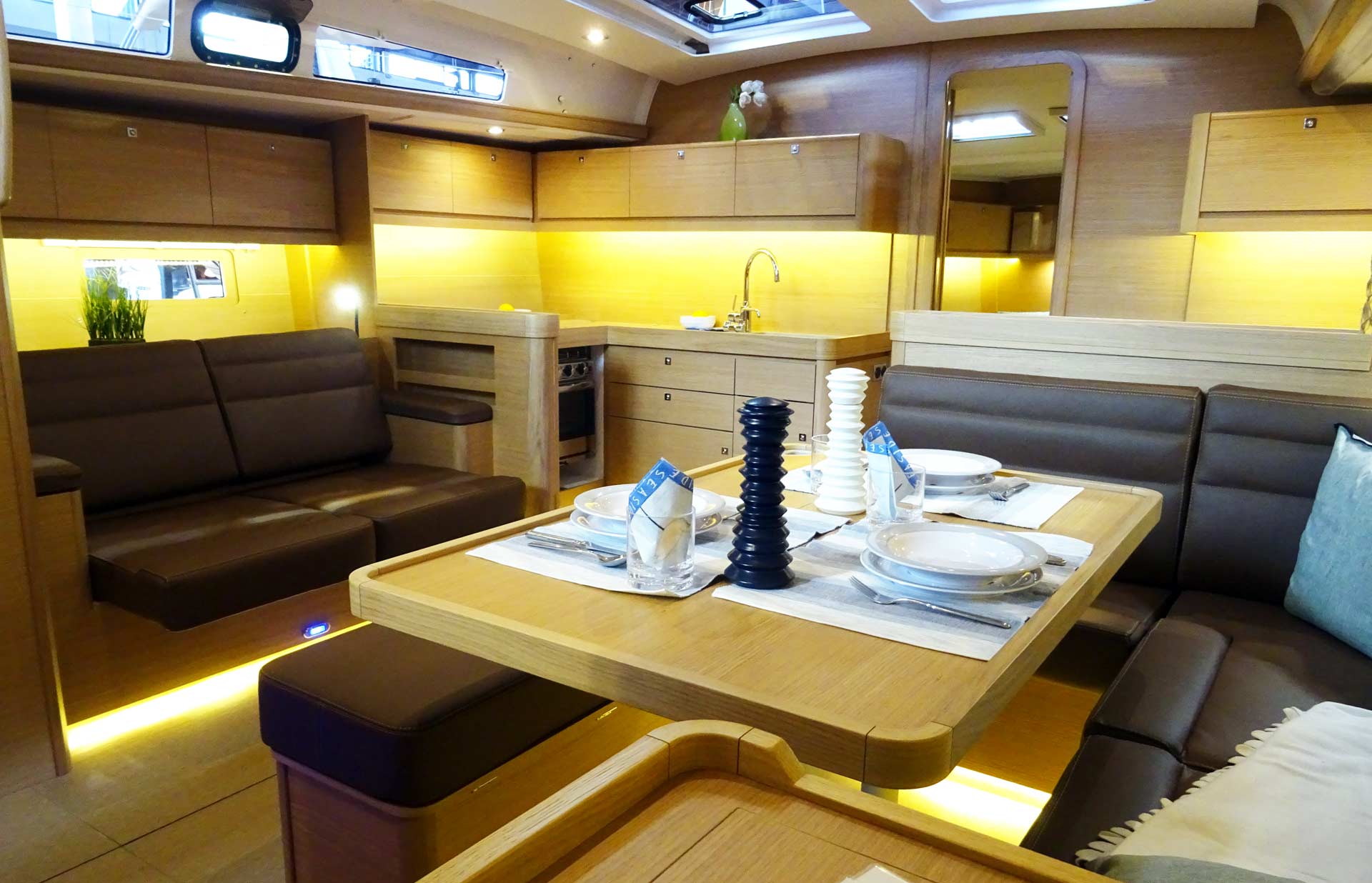The image depicts a cozy and modern interior room, possibly within a high-end private yacht or an upscale RV motorhome. The space is designed with a neutral color palette of cream, tan, gray, and various shades of brown, including blonde wood cabinetry which gives a Scandinavian feel. The focal point is a dining area featuring a booth-style seating arrangement along the edge, with an additional loveseat-sized brown upholstered seat opposite it. The table is set for three, with neatly folded napkins in a glass and a decorative black and white salt and pepper shaker set.

Above, cabinetry lines the room, providing ample storage while also housing under-cabinet lighting that illuminates a sink area in the far left-hand corner, complete with a dishwashing rack. Despite the lack of visible windows, the space is well-lit with overhead and under-cabinet lighting, enhancing its clean and modern aesthetic. The room's thoughtful design elements, such as the possibility of converting the table area into an extra sleeping space, highlight its functionality and elegance.